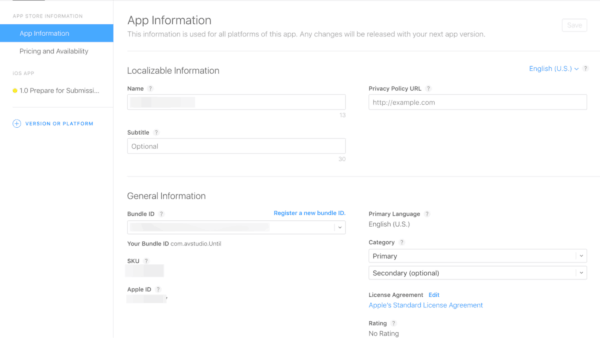The image depicts a detailed, albeit partially obscured, interface from an application submission platform. The page appears to be divided vertically, with a narrow column on the left and a wider section occupying the rest of the page.

**Left Column:**
In the narrow left-hand column, the header reads "App Store for" (the following word is unclear). Below this header is a blue bar labeled "App Information." Further down are sections titled "Pricing and Availability," followed by another indistinct title. There is a yellow-highlighted section labeled "1.0 Prepare for Submission." Beneath this, a circular icon is visible, although the text within it is unreadable, indicating something about a platform.

**Main Document Area:**
In the wider right section of the page, the header in large, bold text reads "App Information." The text below elaborates that this information is used for the platform and that any changes will be released with the next app version. Adjacent to this text, on the right side, is a prominently placed box labeled "Save." Below this is a horizontal line followed by a section labeled "Localized Information."

Within the "Localized Information" section:
- A rectangular box labeled "Name" in bold text appears.
- To the right of this box, there is another box with the label "Pricing Policy URL" in bold text.

Overall, the image showcases an interface related to app submission, detailing sections for app information, pricing and availability, and localizing information, with clearly defined areas for entering the app's name and pricing policy URL.